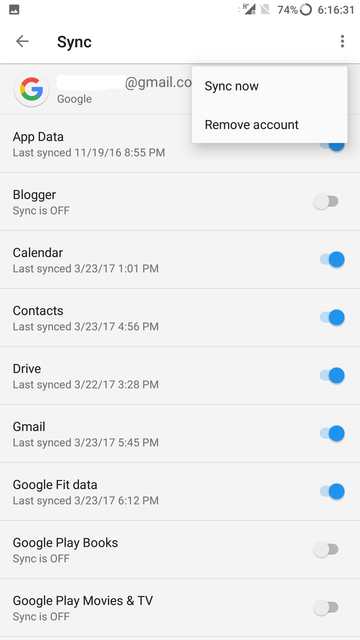Screenshot of a Google Sync Settings Screen:

The screenshot captures the top portion of a mobile device screen, displaying Google account sync settings. At the very top, the word "Sync" is prominently shown, indicating the section the user is in. Below this, a box is visible, providing options to either "Sync now" or "Remove account." Additionally, there is a field to input or view the associated email address.

Further down, a detailed list outlines the synchronization status of various Google services. The following services are enabled for sync: App Data, Calendar, Contacts, Drive, and Gmail. Conversely, Blogger, Google Play Books, and Google Play Movies & TV are disabled. A timestamp indicates that App Data was last synced on November 19th.